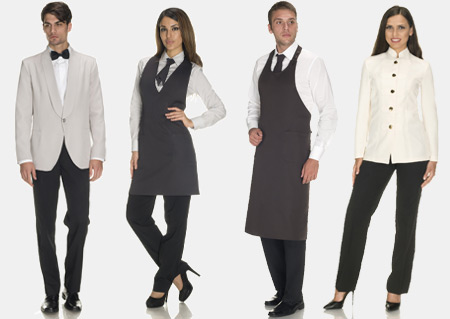The image displays four models, each dressed in uniforms resembling those of high-end restaurant staff, posing in a catalog style. 

On the left, a young man with short brown hair looks down with a sulky expression. He is outfitted in a white or off-white suit jacket paired with a black bow tie, white shirt, and black pants. Beside him stands a young woman with straight brown hair and noticeable makeup. Her ensemble includes a button-up white shirt, adorned with a ribbon or small tie, a tight-fitting black apron, black pants, and high heels.

Next to her is a man dressed in a white shirt and black tie, complemented by a long, black apron and dark pants, suggesting a work role possibly in the kitchen or as a server. Finally, on the far right, a woman with long, straight black hair wears a dressy white chef's coat with black buttons, black pants, and black pumps. The formality and consistency of the outfits hint at roles ranging from kitchen staff to front-of-house employees in an upscale dining establishment.